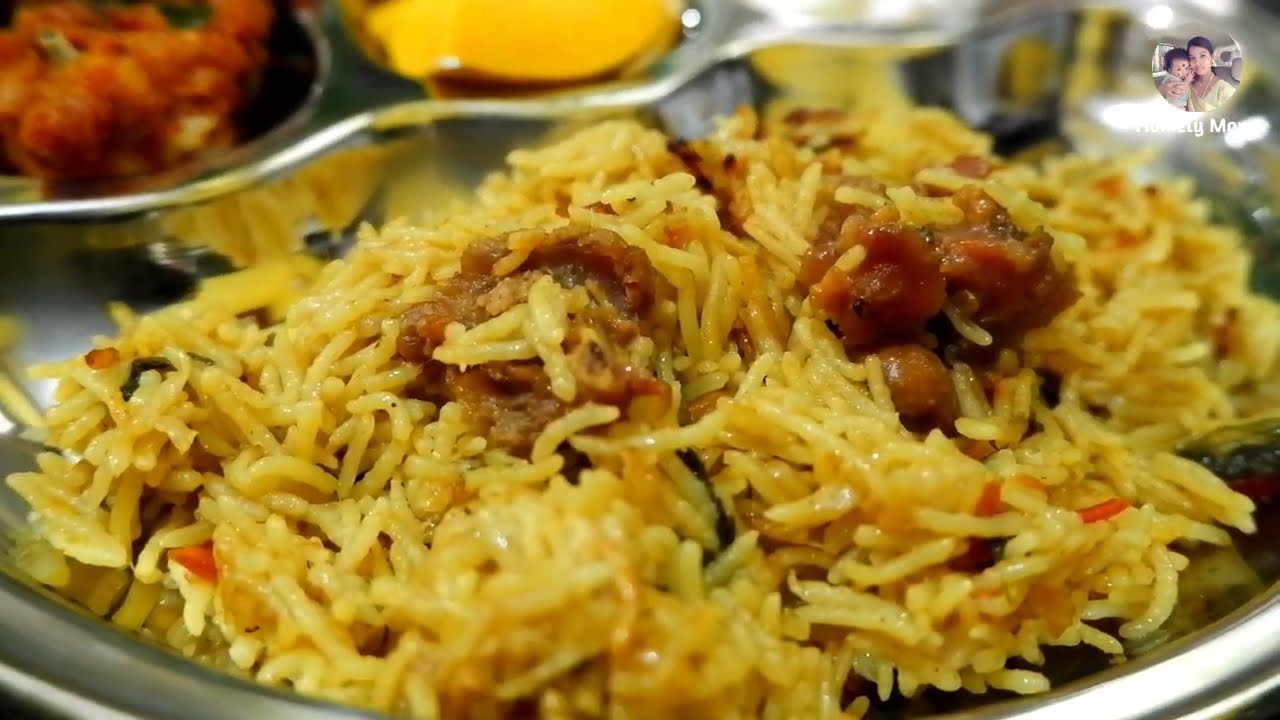The photograph is a detailed close-up of a plate of food, prominently featuring yellow saffron rice. The rice grains are long and distinctly separated, not clumped together, and it appears to be served on a silver metal plate. Among the rice, there are visible chunks of brownish-colored chicken, possibly sesame seed chicken, although not entirely clear. In the background, the image blurs, revealing more food on other plates, including what may be queso or melted cheese and some type of sauce, hinting at a possible Mexican restaurant setting. Additionally, in the upper right-hand corner, there is a small circular profile picture of the individual who posted the photo, accompanied by faint letters that are difficult to discern but suggest the presence of text. The entire image itself is in high clarity, despite the background blur.